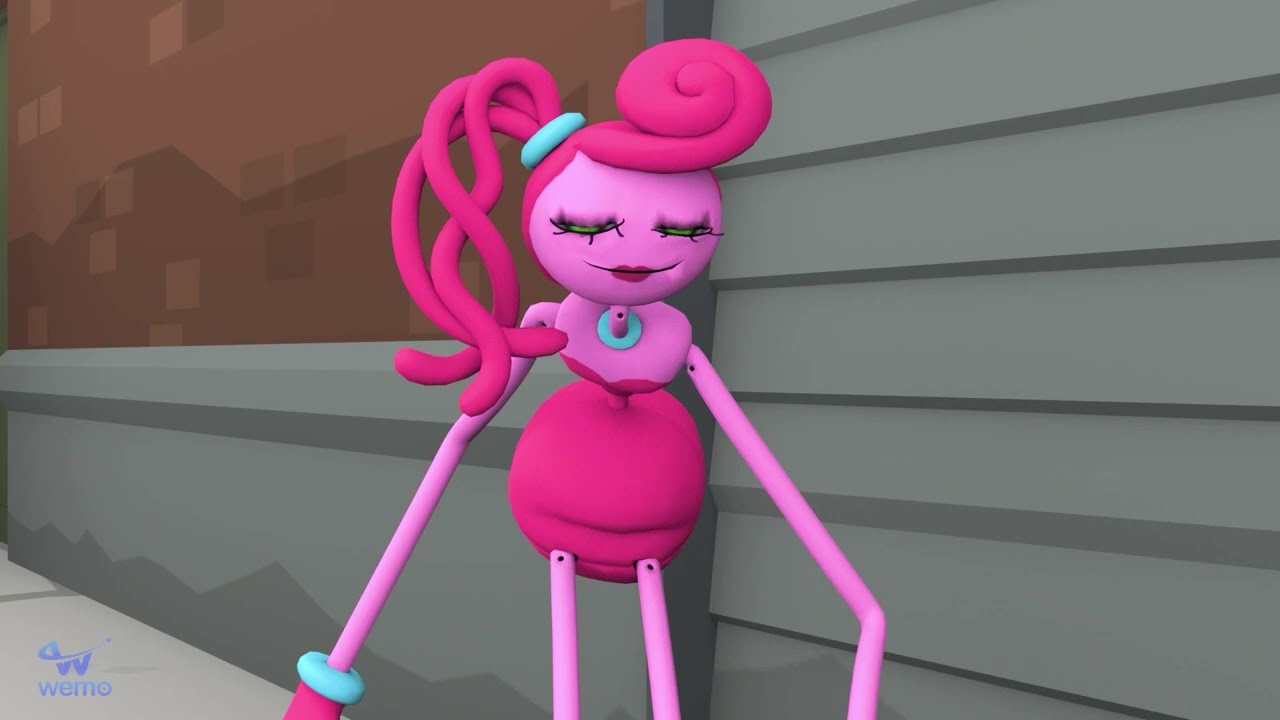The image is a colorful and detailed computer rendering, likely from a game or children's animation. It depicts a pink, ant-like female character with long, slender limbs and segmented, spherical body parts including a thorax, abdomen, and circular head. Her torso and hair are a darker shade of pink, contrasting with her lighter pink skin. She accessorizes with blue items—a hairband, necklace, and bracelets. She has a cheerful expression with nearly shut eyes and a wide smile. The background features a gray wall with a brown panel resembling stacked wooden slats. In the bottom left corner, an abstract, dog-like icon sits above the word "WEMO," which appears twice, suggesting it could be some sort of watermark or branding.